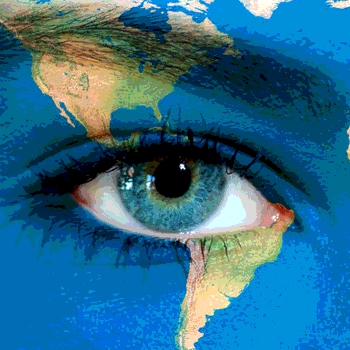This digital image is a small, square artistic portrayal focusing on a single eye and its surrounding area. Dominated by shades of blue, the piece centers on a detailed depiction of a blue eye that contains hints of green near a black pupil, accompanied by whites tinged with pink in the corners. The eye is framed by clearly defined eyelashes and an eyebrow above. The background, primarily blue, is interspersed with varying shades and dotted textures, blending seamlessly behind the focal eye. Dripping from the eye's corner and from above, streaks of tan and greenish-yellow hues add depth and intrigue. Enhancing the abstract nature, the blue areas around the eye subtly incorporate painted representations of continents, with South America positioned below the eye, while the upper part features regions resembling North America, parts of Europe, and China. This artistic blend creates a mesmerizing and visually rich composition.